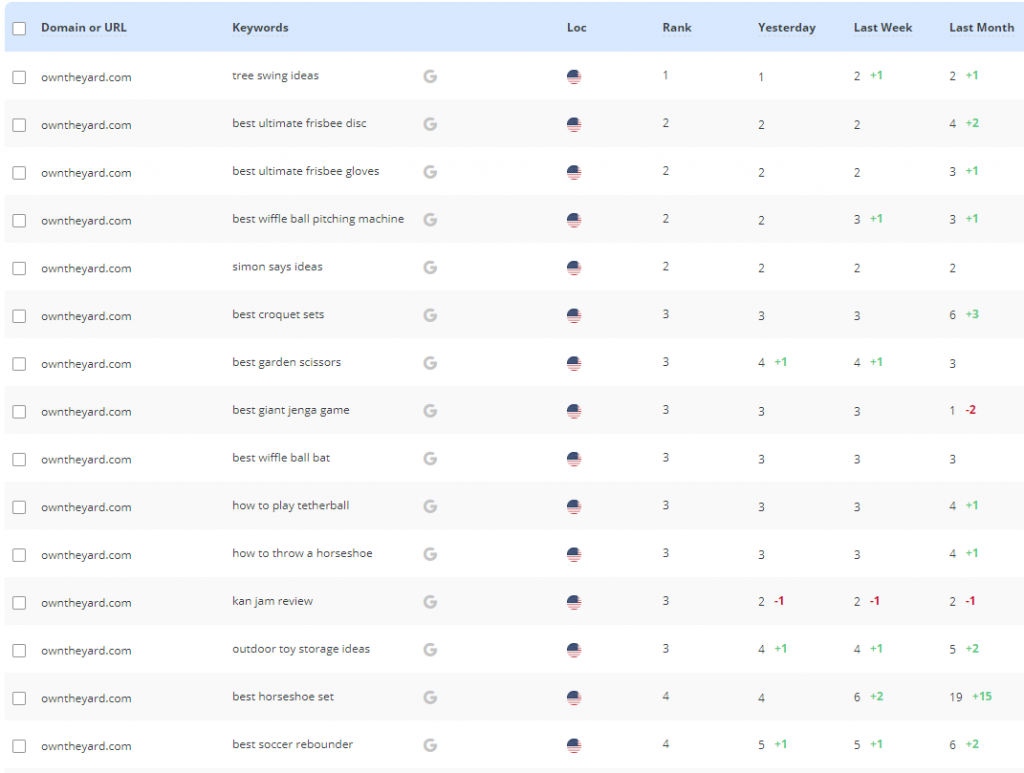The image showcases a detailed analytical page displaying domain performance metrics. At the top, a header bar with a light blue background and dark black font organizes the data into columns labeled: "Domain or URL," "Keywords," "Location," "Rank," "Yesterday," "Last Week," and "Last Month." 

Beneath the header, there are 15 rows that alternate between white and light gray backgrounds. Each row pertains to the same domain, "owntheyard.com," which is displayed in a dark gray font. Following the domain in each row, keywords are listed specific to each URL entry—such as "tree swing ideas" for the first row. 

Each row includes a small Google icon, followed by the location marked by a USA flag. The current rank for "owntheyard.com" is then detailed: today’s rank holds the top position at number 1, matching yesterday’s rank. Last week, the rank was 2, noted with a green '+1' indicator, signifying an upward movement. Similarly, the rank from last month also shows a '+1' improvement from a previous rank of 2.

This pattern of ranking information and movement is consistently repeated across all 15 rows. For each keyword associated with "owntheyard.com," the table meticulously details the current rank, previous ranks, and any changes in rank over the past day, week, and month. Every shift in ranking is highlighted with green markers to easily indicate positive movements.